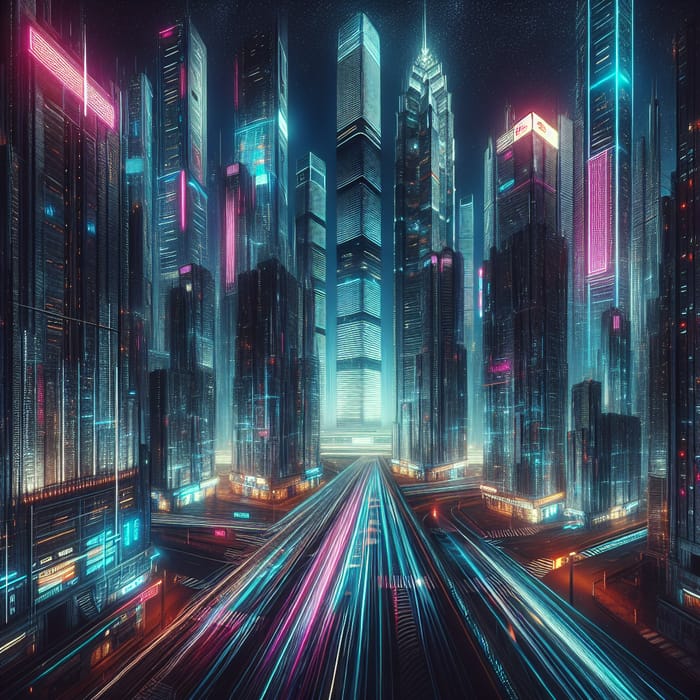The image is a detailed, computer-generated depiction of a futuristic city at night. Dominating the bottom center extending towards the middle is a bustling highway illuminated by vibrant blue and pink light rays, which seem to radiate from the structures beyond. Flanking this highway are numerous skyscrapers, characterized by their sleek black and grey exteriors interspersed with striking pink and purple light accents. These buildings rise tall into the night sky, which is a deep black adorned with subtle specks of white, resembling distant stars. Toward the highway's end stands a remarkably tall and thin building, distinctively patterned with a series of cube shapes. The scene captures a blend of advanced architecture and dynamic lighting, creating a vivid and immersive view of a technologically advanced urban landscape.